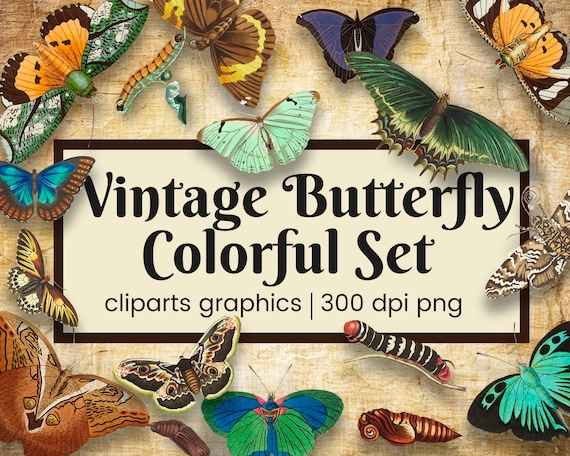This image is a digital advertisement for a vintage butterfly clipart set. The ad features a distressed, brown-tan background with the title "Vintage Butterfly Colorful Set, Clip Arts, Graphics, 300 DPI PNG" prominently displayed in an elegant, older-style black script, framed within a horizontal brown rectangle. Surrounding the central text are various butterflies and caterpillars, showcasing a diverse array of species and developmental stages, including larvae, caterpillars, and adult butterflies. The butterflies come in a rich palette of colors, including bright turquoise, pale seafoam green, aquamarine, purple with orange details, and camouflage patterns. Many butterflies have distinct black patterns and some caterpillars display contrasting stripes. The detailed and colorful arrangement of the butterflies and caterpillars creates a visually engaging and vibrant composition.